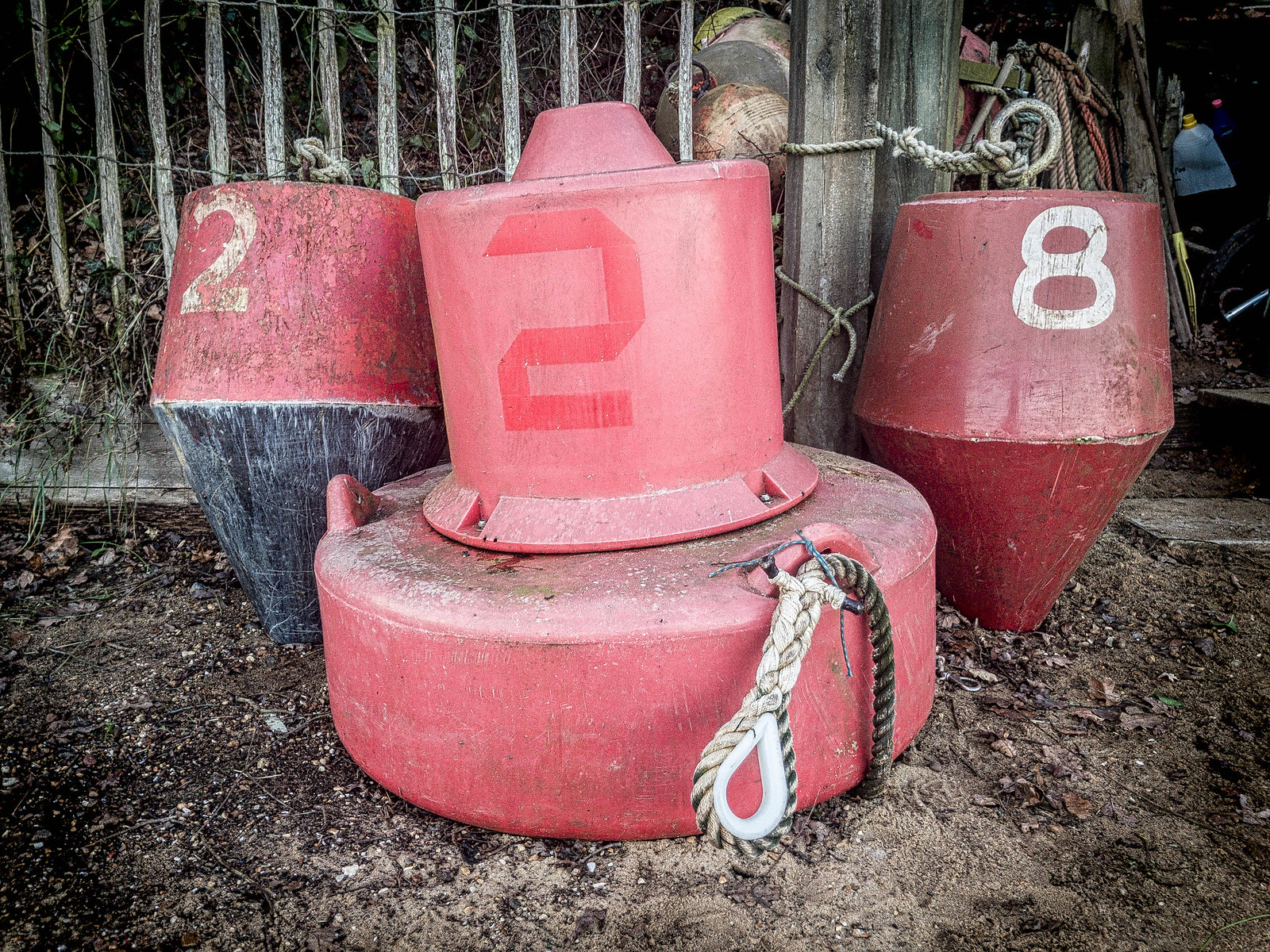This desaturated color photograph captures a scene dominated by three prominently displayed buoys leaning against a weather-worn, greyish metallic fence, with some greyed-out vegetation poking through. The central focus is on a large red buoy, consisting of a rounded, drum-like base with a larger red cylinder and a smaller top, all seemingly part of the same object. This buoy features a red number "2" and has a white rope threaded through a metal hook on its right side. To the left of this central buoy lies another buoy with a distinct shape; it features a red top and a lower black, pointed section, resembling a pencil tip. This left buoy also bears a faded white number "2". On the right side of the central buoy is the third in the row, entirely red with a similar cylindrical shape and pointed bottom, marked with a white number "8". All buoys appear to be anchored to the fence behind them, which looks old and worn. Additional items, possibly other buoys, balls, and maybe even a paddle, are visible behind the fence along with something blue in the upper right corner of the image whose identity remains unclear. This collection of weather-beaten marine buoys and related equipment, set against the backdrop of the aged fence, suggests a storage spot near a dock or beach.